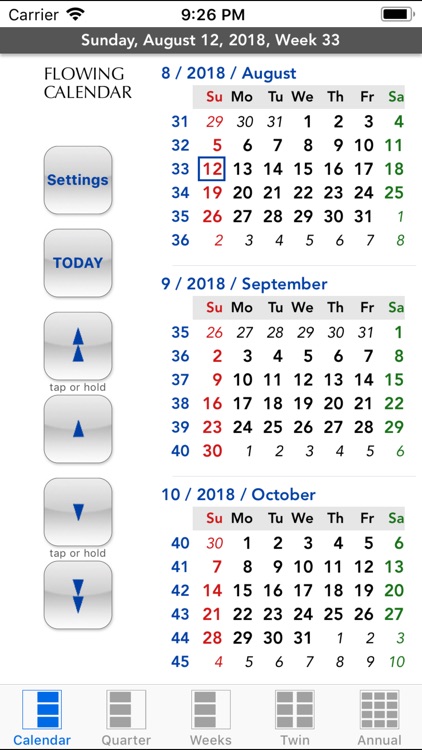The image is a detailed screenshot of a mobile application or website with various sections and buttons related to a calendar function. 

At the very top, there is a white border, alongside a black notification bar displaying standard mobile indicators. On the left-hand side, it reads "Carrier" and shows a fully filled, upside-down triangle Wi-Fi signal in black. Centered at the top, the time is displayed as "9:26 PM," typical of a mobile device interface. To the right, a battery icon indicates a 95% charge.

Directly underneath, there's a dark grey strip with the current date in white text: "Sunday, August 12th, 2018, week 33."

The main section of the page is divided into two parts. On the left side, the section is titled "Flowing Calendar." Below this, there are several grey gradient buttons (grey at the top fading to white at the bottom) with blue text. The first button is labeled "Settings," the second "Today," and the third contains two blue triangles stacked vertically. Below these, more buttons follow: one with an upward-facing triangle, another with a downward-facing triangle, and a third with two downward-facing triangles. Each button has "Tap or Hold" written beneath it in small letters.

On the right side of the page are multiple calendar views. The first calendar section is labeled "8/2018/August," with the date "12" highlighted by a box. Below it, there are calendars for September ("9/2018/September") and October ("10/2018/October").

At the bottom of the page, there are options for different calendar views:
1. "Calendar" with an icon showing three rectangles inside a square, all in blue.
2. "Quarter" with a similar icon but all in grey.
3. "Weeks" with the same icon configuration as "Quarter" in grey.
4. "Twin," represented by a square filled with six rectangles, in grey.
5. "Annual," depicted by a square with three small rectangles across and four downward, also in grey.

Each of these icons corresponds to different calendar display modes, allowing the user to choose how they wish to view their calendar.